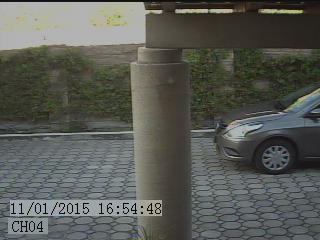This image appears to be a still shot from a security camera, captured on November 1, 2015, at 16:54:48, as indicated by the digitized timestamp in the lower left corner. The camera seems to be positioned outdoors, possibly at the front of a house or a hotel driveway, as suggested by the layout and elements visible in the frame. The central feature of the image is a thick, beige stone or concrete pillar, supporting an overhang with horizontal wooden slats extending across it. The driveway is paved with gray, octagonal or circular tiles. In the top right of the image, the front end of a gray, possibly brownish or drab-colored sedan is visible, with its headlights on, partially cut off at the driver's side door. In the background, a brick wall covered in dark green ivy stretches across the scene, contributing to the somewhat muted and drab appearance of the overall image.